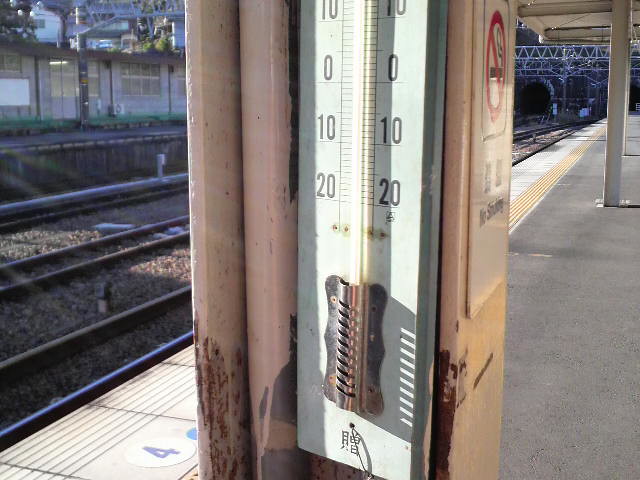The image depicts a bustling train station. On the left-hand side is a yellow platform with a prominent yellow circle marked by a black number "4". Adjacent to this circle, there's a partially visible blue semicircle cutting off the edge of the platform. Ahead, numerous train tracks stretch into the distance. The first set consists of dark brown bars, while the next consists of slightly elevated brown bars. Between these tracks, patches of dirt are visible.

Further down, another set of wooden tracks touches the ground before another dirt-filled gap appears. Beyond these tracks, a gray pole stands tall, surrounded by a brown and green area, seemingly another part of the platform or a pathway. 

To the right, there's a building with a dull gray facade. In the foreground, attached to a distressed beige pole marked with brown streaks, is a detailed thermostat. The thermostat features numbers at the bottom - "20", "10", "0", and another "10" above it, all encased in white and accented with a metal piece at its base. Asian symbols grace the bottom of the thermostat, though their meaning remains unclear. Tied to this same pole is a no smoking sign, framed by a black outline, a vivid red prohibition symbol, and a black cigarette graphic at its center.